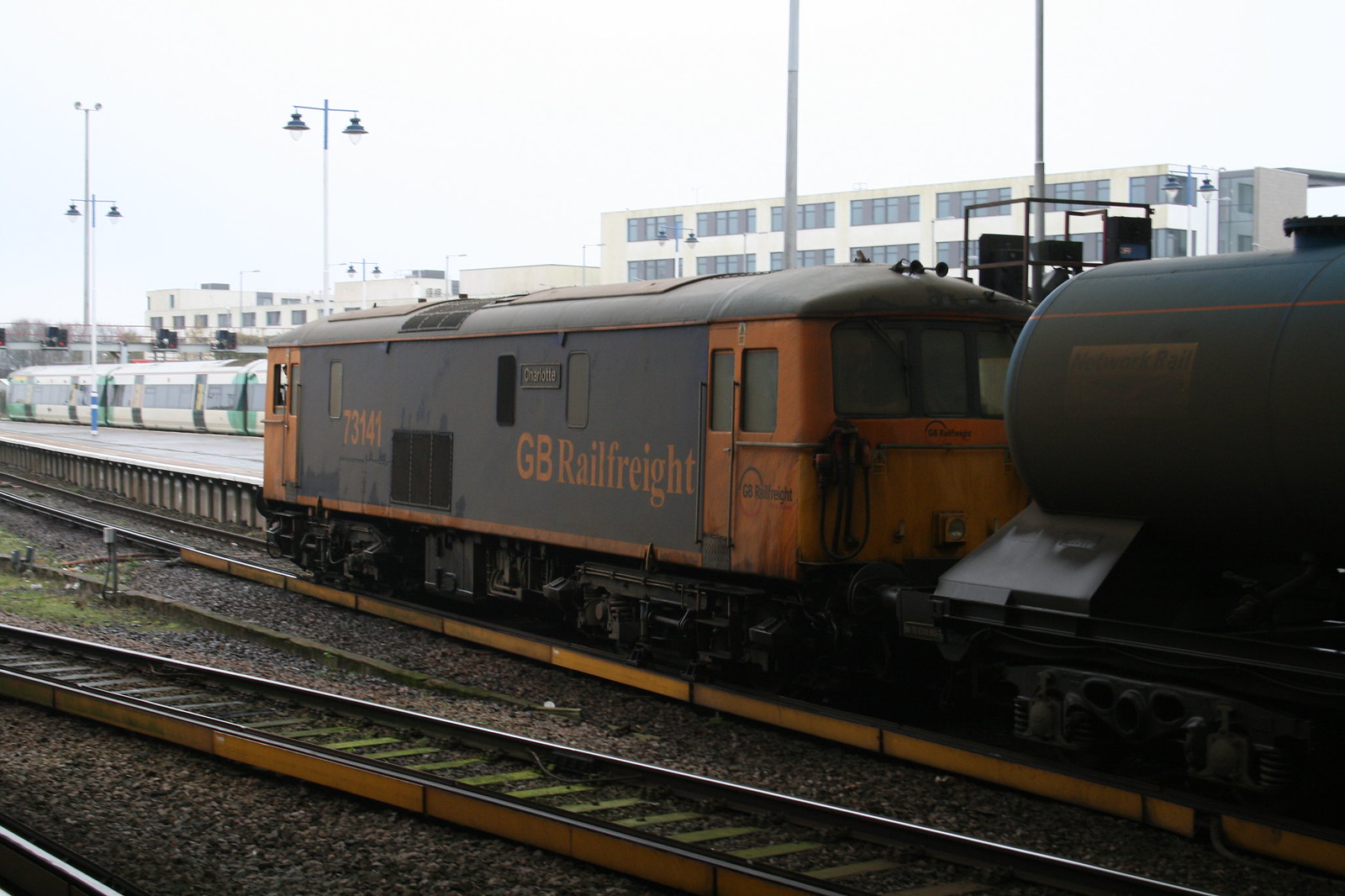The image depicts an urban train yard with multiple sets of tracks in the foreground. The ground under the tracks is covered in dark brown gravel. The tracks stand out with their yellowish sides. Centered in the image is a predominantly black train emblazoned with "GB Rail Freight" in orange letters, bearing the number 73141. In front of this train, there's a black tanker car with a thin orange stripe. In the background, a commuter train, colored white with green trim, is visible. Additional elements in the scene include lighting posts on metal towers and office buildings with white and cream facades, which feature numerous windows. The scene is set under an overcast, light grayish-blue sky, indicating daytime.